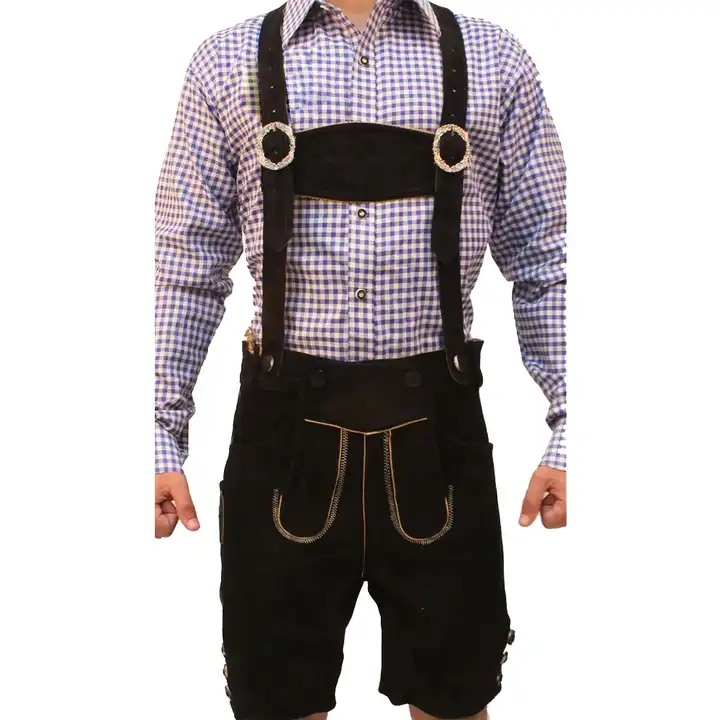The photograph depicts a Caucasian man with pale skin, shown from neck to knee level, standing against a white background. He is wearing a traditional lederhosen outfit, which includes black suspenders with two circular, silvery buckles near the chest area. These suspenders connect to black shorts that cut off just above the knee. His shirt is a long-sleeve button-down with a blue and white plaid pattern and a collar. The man's stance is relaxed, with his arms down and fists partially visible. The outfit's details also include additional black buttons around the waist area.